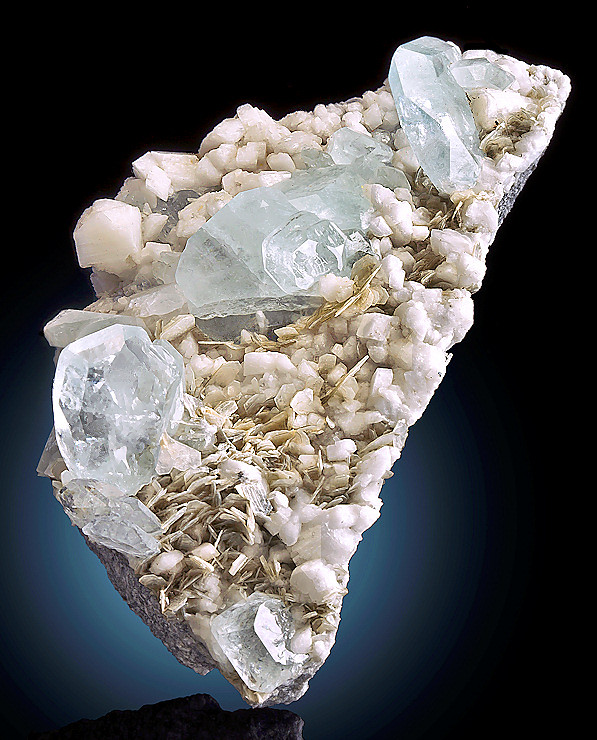This image features a striking rock structure, prominently showcasing a large, nearly triangular rock adorned with various stones and crystals. The main rock appears to be cracked open, revealing intricate layers that house cream-colored pebbles and larger, shiny stones reminiscent of ice cubes. The structure is artistically arranged, appearing almost impossible as it seemingly balances on a fine point atop a darker, black rock.

Some of the stones embedded within the primary rock are translucent, giving a crystalline quality, while others remain solid white, lending a stark contrast in texture and color. The overall composition reveals a jagged, half-circle form at the base, with ascending crystals emerging from it. Suspended and meticulously placed, this rock sculpture likely resides in a museum or gallery setting.

The backdrop enhances the sculpture's visual impact with a gradient of blue at the bottom, transitioning to black towards the top and right side. This dramatic background highlights the crystalline forms and provides depth to the entire composition.